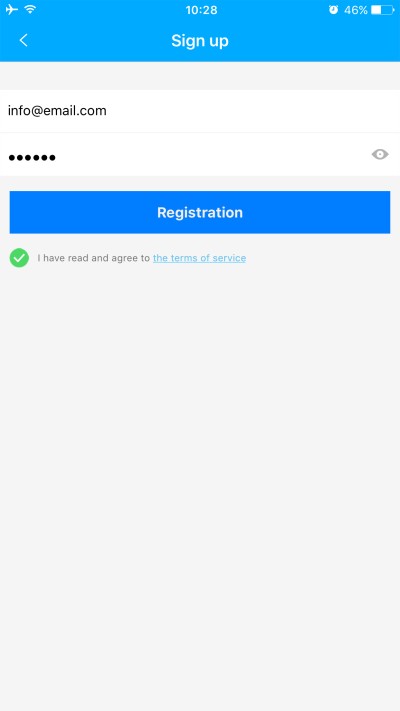This portrait-oriented image, roughly the size of a cell phone screen, captures a sign-up page characterized by a minimalist design. The top 40% of the image features all the essential elements, while the remaining 60% is a plain light gray background.

At the very top is a light to medium blue header, spanning the width of the image. In the upper left corner, three small white icons are aligned: an airplane, a Wi-Fi symbol (resembling a slice of pizza with three lines), and an alarm clock. Centrally placed at the top, the time reads "10:28," and to the right, a battery icon indicates a 46% charge, accompanied by the numeric "46%".

Below the top header is a navigational row within the blue field. On the left side, a left-facing arrow is visible, and centrally, bold white text reads "Sign Up".

The rest of the image transitions to a light gray background. Immediately beneath the blue header sits a narrow gray strip. Below this, two white fields span the image’s width, separated by a thin gray line. The top field contains left-justified text that reads "info at email.com." The field below displays six black dots, symbolizing a hidden password, with an eye-icon to the far right, offering the option to reveal the password.

Further down, a darker medium blue rectangle is centered, slightly narrower than the full width of the image, bordered by gray on both sides. In the center of this rectangle, "Registration" is written in white, center-justified text.

Directly below this, a green circle with a white checkmark signifies an agreement statement. Beside it, dark gray text reads "I have read and agreed to the terms of service," with "terms of service" highlighted in a clickable, underlined light to medium blue.

The bottom portion of the image is a continuation of the plain light gray background, completing the rectangular composition.